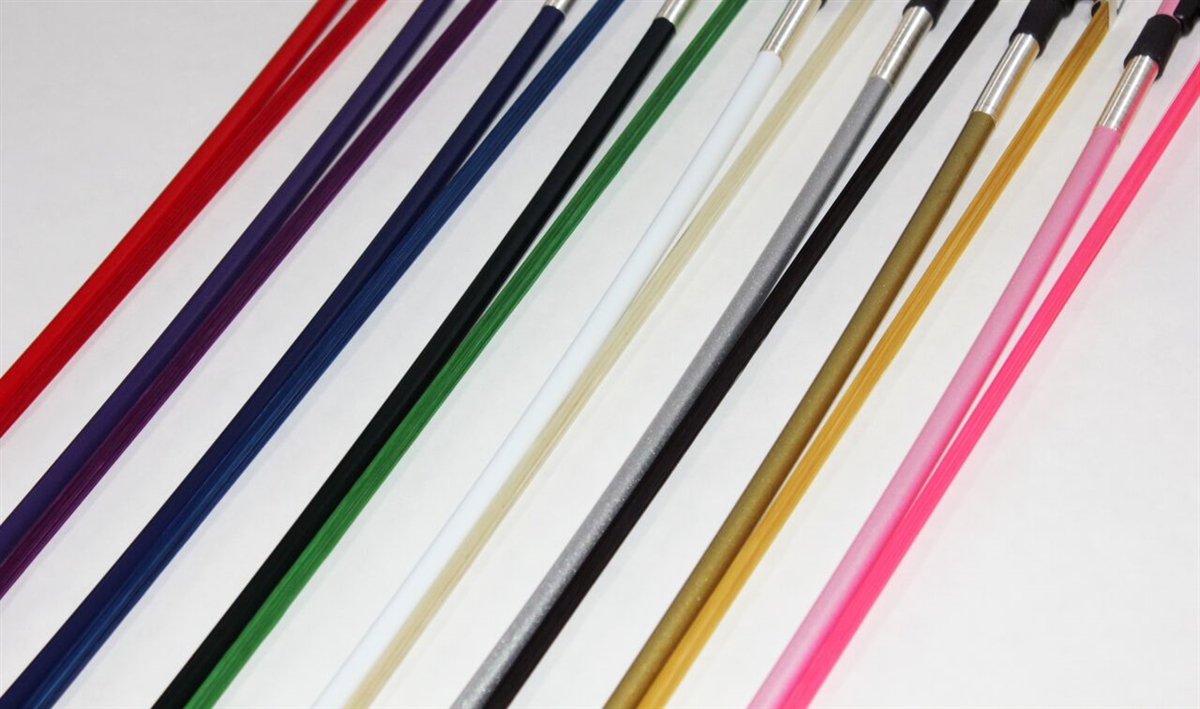This photograph depicts an orderly arrangement of various colored laces lying vertically side by side on a white background. Each lace is paired with a corresponding painted line that matches its color. The colors included are red, several shades of blue including navy, multiple shades of black, green, white, gray (silver), brown (khaki), mustard, light pink, dark pink, and purple. The laces, which appear to be similar to ropes or possibly pointers or batons, are bound at one end with silver wiring and capped with a black tip. The layout is highly organized, with each lace neatly placed about an inch apart from the next, emphasizing the color coordination and meticulous alignment.